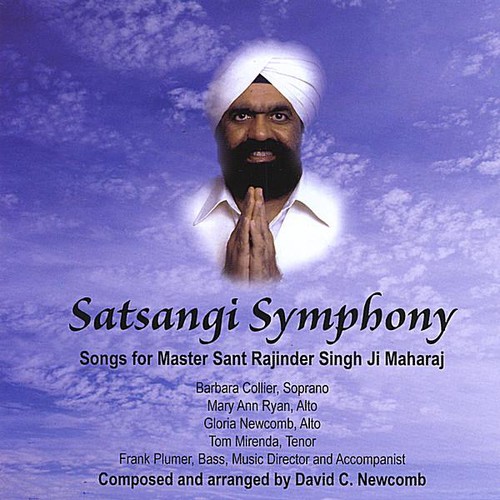The image is likely an album cover or an event poster. The background features a purplish-blue sky with multiple translucent clouds. In the top half, there's a central circular photograph of an Indian man with thick black eyebrows, brown eyes, a black beard, and a mustache. He is wearing a button-up white shirt along with a white vest and a white turban, though the top of the turban is cut off from the image. The man has his hands together in a prayer motion.

Below this central image, black text covers most of the bottom half. The text prominently reads, "Satsangi Symphony." Followed by, "Songs for Master Sat Rajinder Singh Ji Maharaj." Underneath, vertically listed are the names and roles of people involved in the symphony: "Barbara Collier, Soprano; Mary Ann Ryan, Alto; Gloria Newcomb, Alto; Tom Marendo, Tenor; Frank Plumer, Bass; Music Director and Accompanist." At the very bottom, it states, "Composed and Arranged by David C. Newcomb." The overall color palette includes shades of purple, white, gray, and black, contributing to the serene and reverent tone of the image.